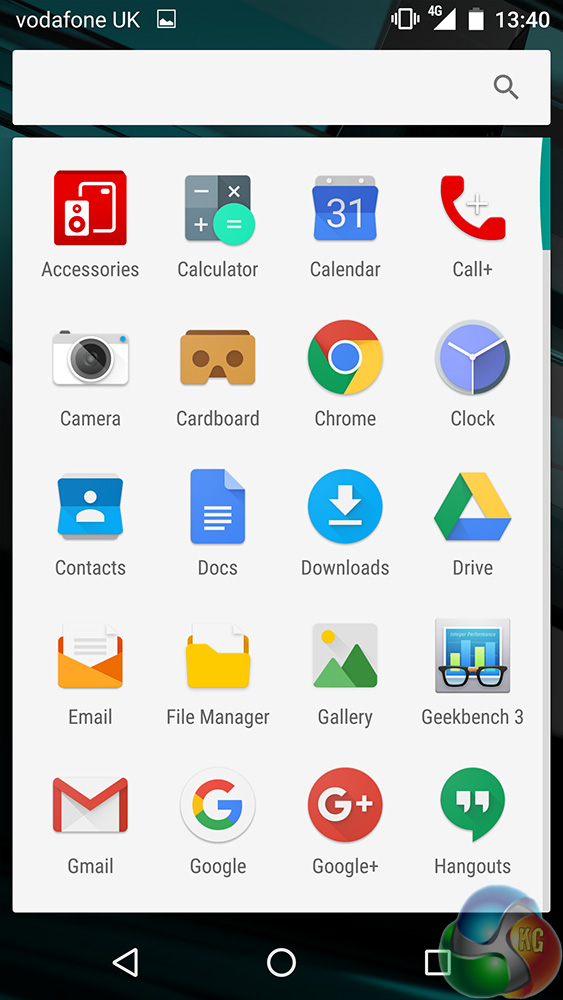This is a detailed screenshot of a Vodafone UK smartphone interface. The entire screenshot has a vertical rectangular black frame. At the top of the screen, there's a black bar displaying the Vodafone UK carrier name on the top left corner, with battery status and current time (13:40 in military time) on the top right. Just below this status bar, there's a search bar featuring the iconic magnifying glass symbol on the right side, allowing users to search through their device.

Beneath the search bar, there's a large gray rectangle showcasing the app drawer, which reveals a list of installed applications. Visible apps include 'Accessories,' 'Calculator,' 'Calendar,' 'Camera,' 'Chrome,' 'Downloads,' 'Documents,' 'Gmail,' 'Google Drive,' 'Gallery,' 'Google+,' and 'Hangouts,' among others. This screenshot captures the moment when the user has unlocked their phone and accessed the app drawer, getting ready to select an application to use.